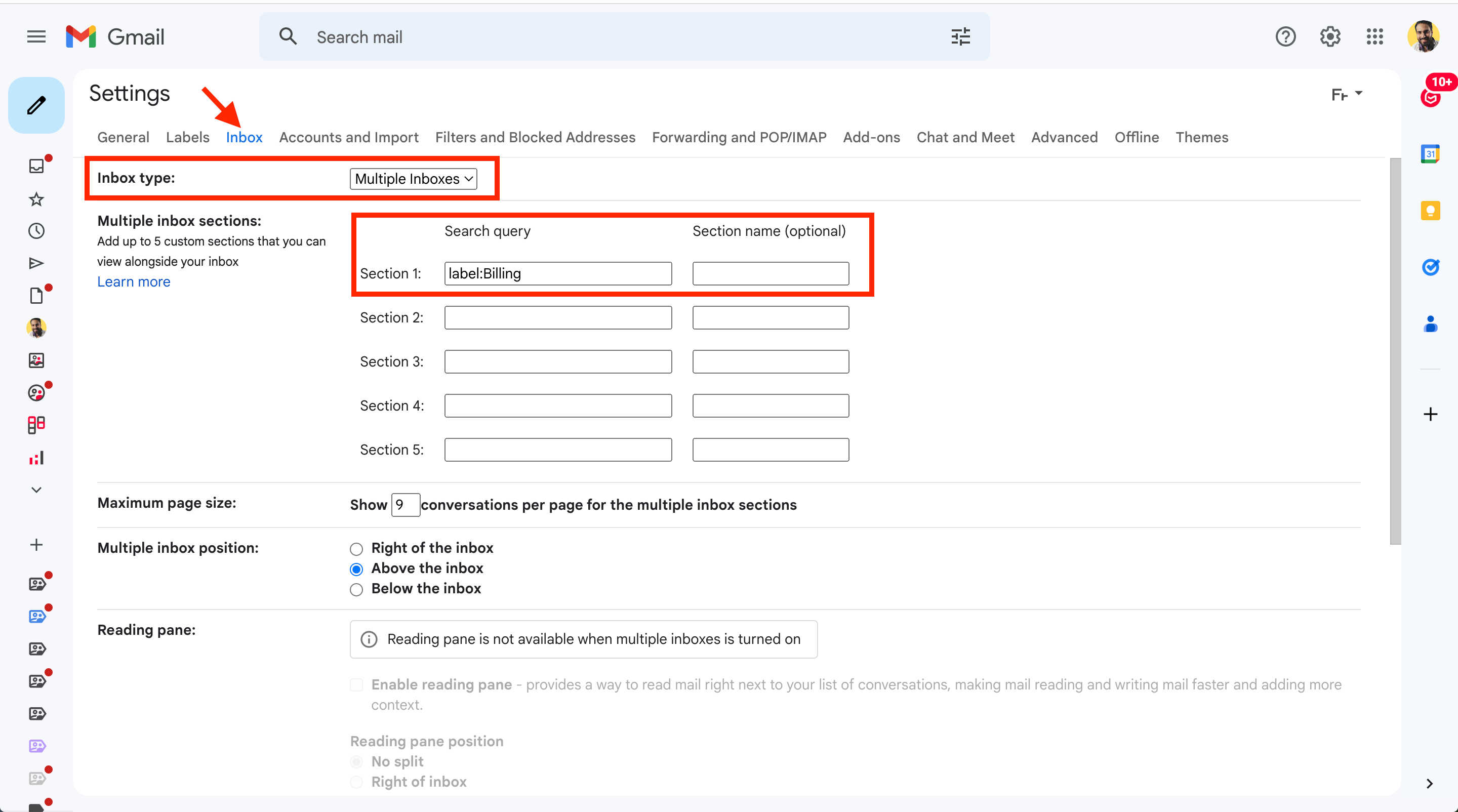The interface showcased here is the Gmail website with a specific focus on its "Settings" and "Multiple Inboxes" configuration. 

In the top left corner, there are three horizontal lines, which act as a menu icon. The word "Gmail" is displayed next to the iconic "M" letter in Google’s colors. Directly to the right is a light blue search bar with the placeholder text "Search Mail." On the far right of the screen, there is a small profile picture of a man against a yellow background. Next to the profile image, there is an icon grid (representing Google Apps), the Settings gear icon, and a question mark in a circle for help.

On the left-hand side, a black heading reads "Settings," followed by a list of categories in gray: General, Labels, Inbox, Accounts and Import, Filters and Blocked Addresses, Forwarding and POP/IMAP, Add-ons, Chat and Meet, Advanced, Offline, and Themes. A red arrow is pointing to the word "Inbox," highlighted in blue to indicate it is currently selected. 

Beneath this "Inbox" setting, the main section reads "Inbox" in black text, enclosed in a red marker box. To the right, there is an option labeled "Multiple Inboxes," which can be clicked to change the setting. Below, it says, "Multiple Inbox Sections - add up to five custom sections that you can view alongside your inbox," with a blue "Learn More" link for additional information.

Further down the screen, there are input fields for "Search Query and Section Name" (marked as optional), comprising Section 1 through Section 5. Each section has two input fields for customized labels, highlighted with a red box around Section 1, which contains the text "label:billing." This suggests it filters emails related to billing. The other sections remain empty.

Additionally, on the left, "Maximum Page Size" is specified with the option to show up to '9' conversations per page in the multiple inbox sections. Below this, "Multiple Inbox Positions" allows users to place the sections "Above the inbox," "Below the inbox," or "Right of the inbox," with the "Above the inbox" option checked in blue.

The "Reading Pane" section is next, containing a banner with the note that it is "not available when multiple inboxes is turned on." In gray text, it explains that enabling the Reading Pane allows for quicker mail reading and writing due to its placement next to the list of conversations.

Lastly, there's the "Reading Pane Position" setting, where you can select either "No split" or "Right of inbox." On the very far left of the screen there is a column of small icons, and on the far right, there’s a small circle icon indicating "10+” alongside several functionality icons.

This detailed setup view captures the complexity and customization options available in Gmail’s "Multiple Inboxes" settings.